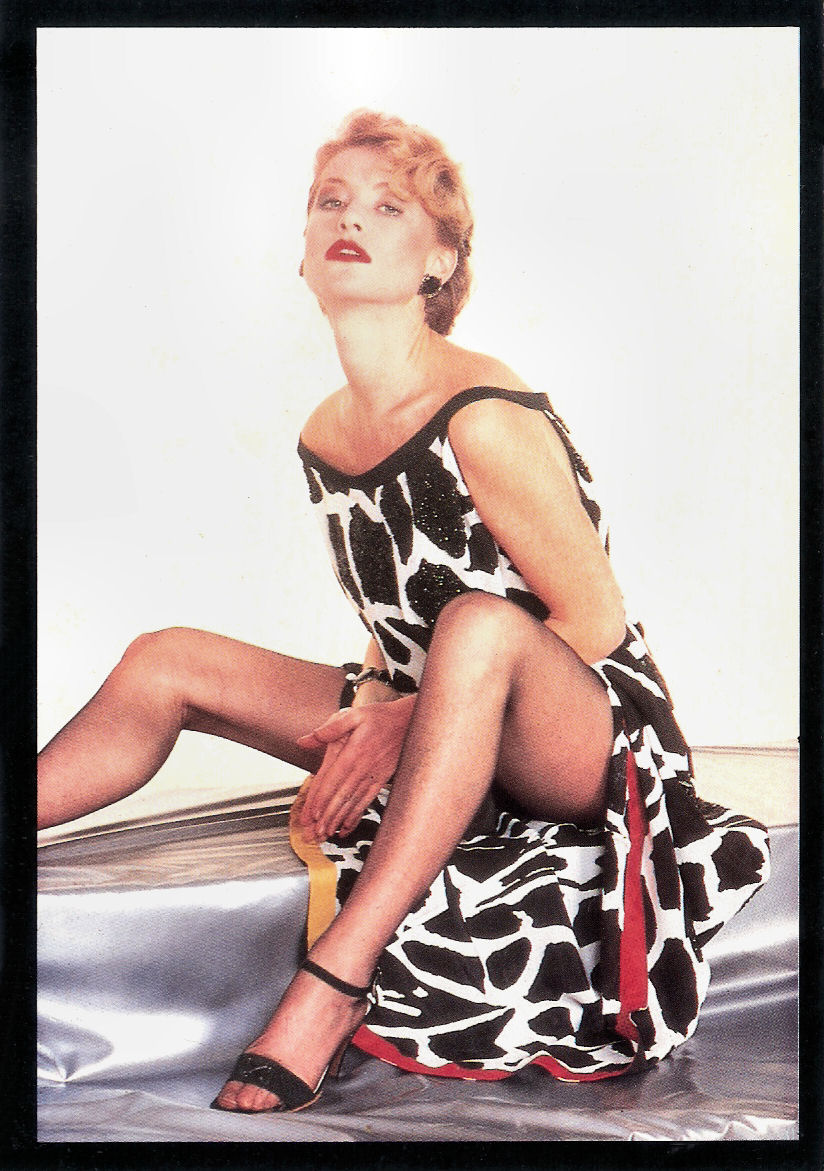This professional photograph captures a poised white woman with short blonde hair and light-colored eyes, seated on a slightly raised, long, silver object adorned with shiny, silver fabric. She is the focal point of the image, centrally positioned against a plain white background and framed by an all-black border. The woman, with bright red lipstick and large black circular earrings, exudes elegance in her black and white cow-pattern dress. Her black high heels, featuring both toe and ankle straps, add to her stylish appearance as one foot rests on the ground and the other extends out of the frame. The indoor setting and the meticulous arrangement of colors—black, white, red, silver, and gray—enhance the professional and polished atmosphere of the photograph.